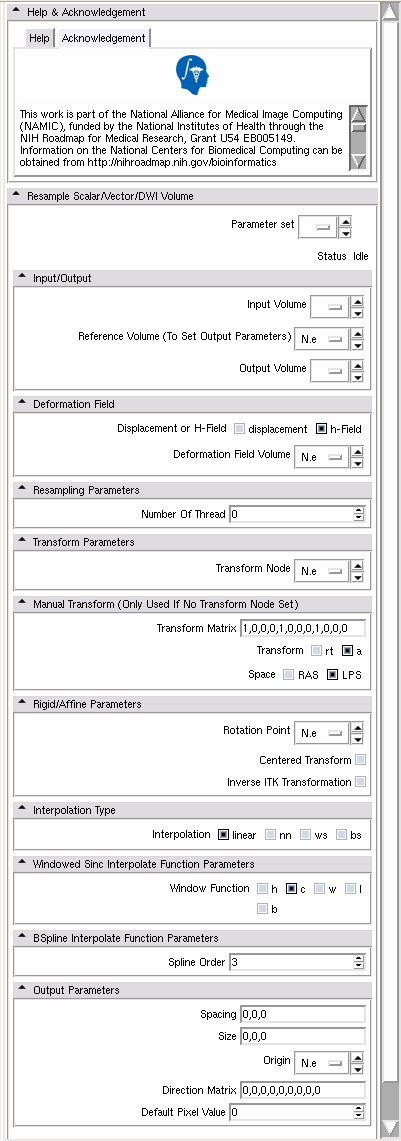The image is a screenshot captured in portrait format, titled "Help and Acknowledgement" at the top. Below this title, there are two tabs labeled "Help" and "Acknowledgement," with the "Help" tab currently open. In the Help section, there is an icon of a blue human head featuring an integral sign and a medical symbol, which appears to be a logo.

Beneath the icon, the text reads: "This work is part of the National Alliance for Medical Image Computing, funded by the National Institute of Health through the NIH Roadmap for Medical Research, grant U54EB005149. Information on the National Centers for Biomedical Computing can be obtained from," followed by an email address that is somewhat hard to read or possibly a website URL.

Further down, the text lists various elements and parameters related to medical imaging:
- "Resample"
- "Scalar"
- "Vector"
- "DWI Volume"
- "Input and Output"
- "Deformation Field"
- "Resampling Parameter"
- "Transform Parameters"
- "Manual Transform (Only Used if No Transform Node Set)"
- "Rigid"
- "Affine Parameters"
- "Interpolation Type"
- "Windowed Sync Interpolate Function Parameters"
- "B-Spline Interpolate Function Parameters"
- "Output Parameters"

The list covers a comprehensive range of settings pertinent to medical image computing and processing.